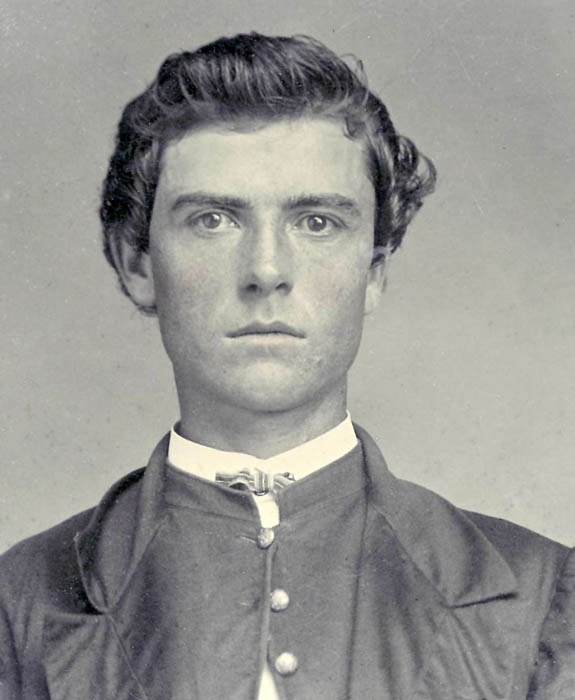The image is a black-and-white photograph of a young man, possibly taken in the late 1800s or early 1900s. The man, identified as Buffalo Bill Cody, is looking straight at the camera with a neutral, almost piercing expression. He has short, dark hair that is pulled back, giving the appearance of either being swept into a bun or ponytail. His attire is quite detailed; he wears a button-up collared coat with ornate, silver or brass buttons, of which three are visible, and only the top button is fastened. Over this, he dons an open black coat and underneath, a high-collar white shirt complemented by a small striped bowtie. His clean-shaven face adds to his youthful appearance. The overall mood of the photo is solemn and reflective, capturing the essence of the era it represents.